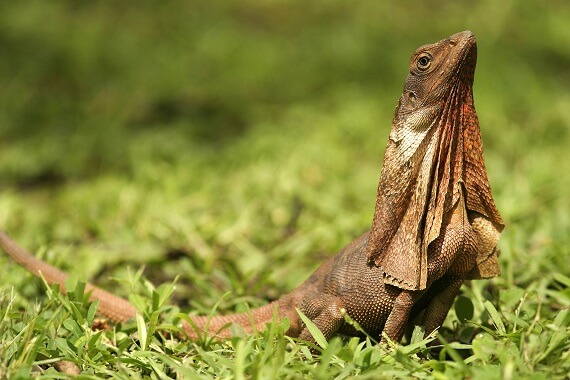In this detailed photograph taken at ground level, a brown reptile, likely a bearded dragon, is set against a lush, green grassy background. The reptile, prominently situated in the foreground, has a distinctive long tail that stretches from the left edge to the center of the image. Its skin, a mix of browns and orangey-red hues, features a leathery texture with loose flaps draping down from its elongated neck. One blue-gray eye, with a black pupil, can be seen clearly as the reptile gazes skywards. The grass in the immediate foreground is crisp and vibrantly green, while the background grass gradually becomes blurred, creating a natural depth effect. The scene is warmly illuminated by morning light, suggesting a clear day, which casts a gentle glow on the grass and the reptile itself.